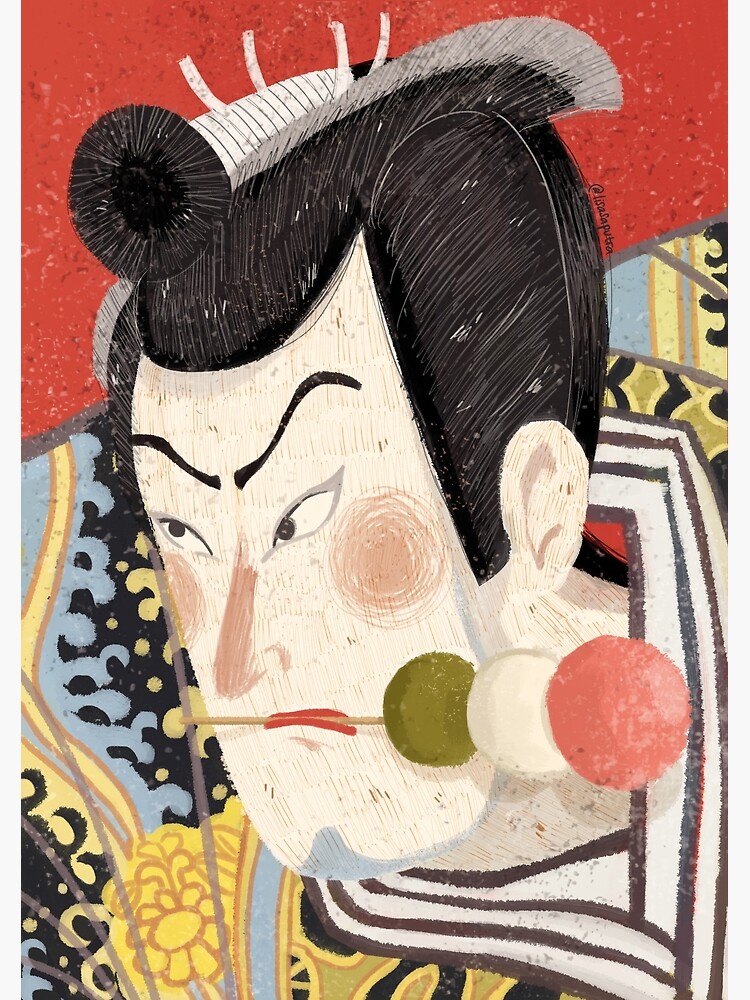The image depicts an Asian-inspired cartoon illustration of a stern-looking woman, characterized by a masculine touch. She has a rather boxy face with very white skin and striking black hair styled in a bun at the front of her head. Her eyebrows are scrunched, contributing to her angry expression. Adding to her distinctive appearance are pink, rosy circles on her cheeks, symbolizing blush. In her mouth, she holds a wooden skewer with three colorful dango balls, a Japanese dessert, featuring a dark green ball, a white ball, and a dark pink ball. The background showcases a red area around her head, transitioning into a tribal print of light blue and yellow waves below her neck, alongside yellow flowers at the base. She is adorned in black, blue, and gold clothing, adding to the rich detail of the illustration.